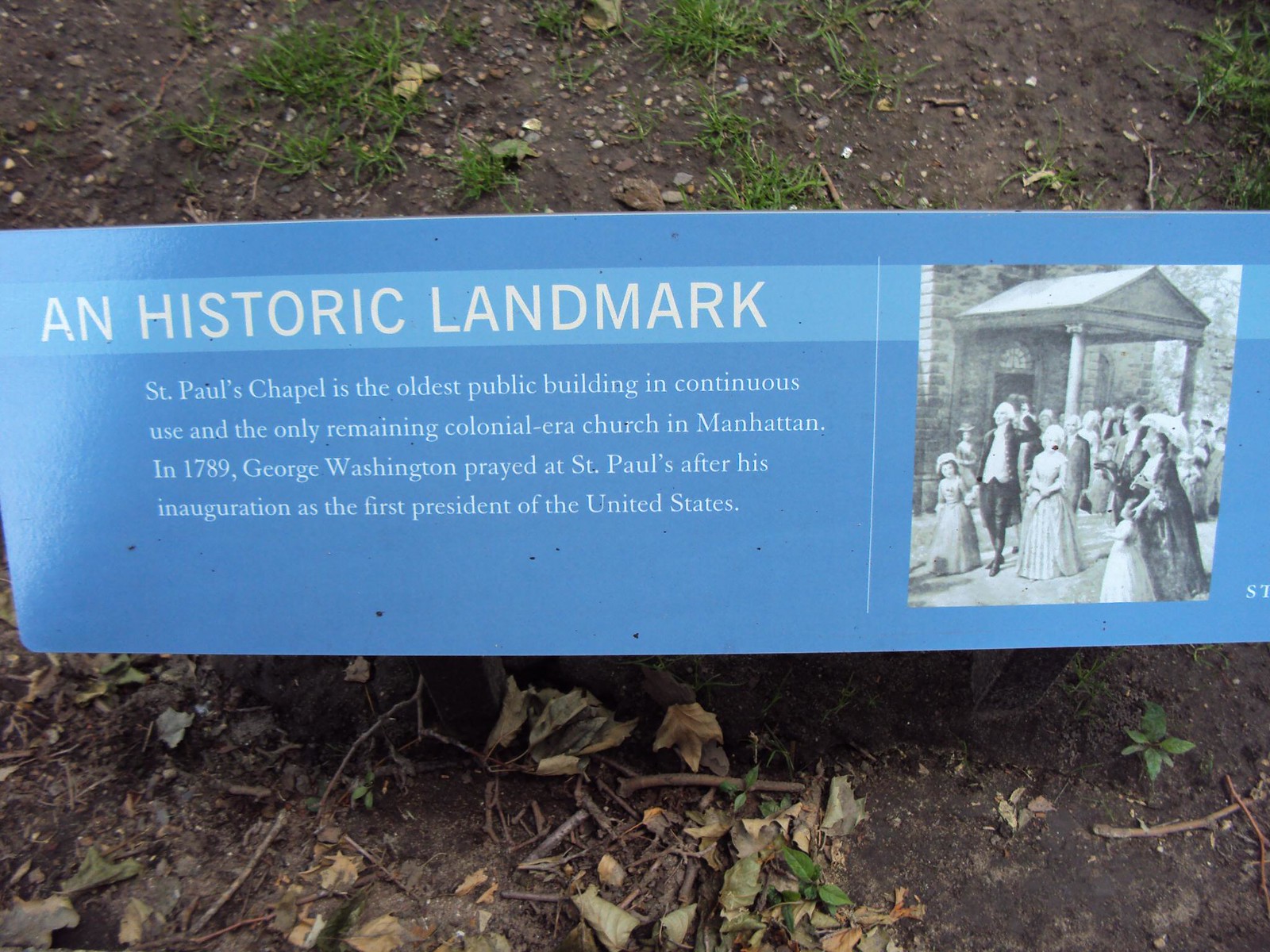The image depicts a rectangular memorial plaque set on the ground, surrounded by patches of earth, dried leaves, and a few green plants. At the top edge of the scene, some grass is visible. The plaque itself has a blue background and features a black and white photograph on its right side. The photograph shows a building with several people standing in front of it, including men, women, and a few girls. The women in the photograph are wearing dresses. The inscription on the plaque identifies it as a historic landmark, stating: "St. Paul's Chapel is the oldest public building in continuous use and the only remaining colonial-era church in Manhattan. In 1789, George Washington prayed at St. Paul's after his inauguration as the first president of the United States."